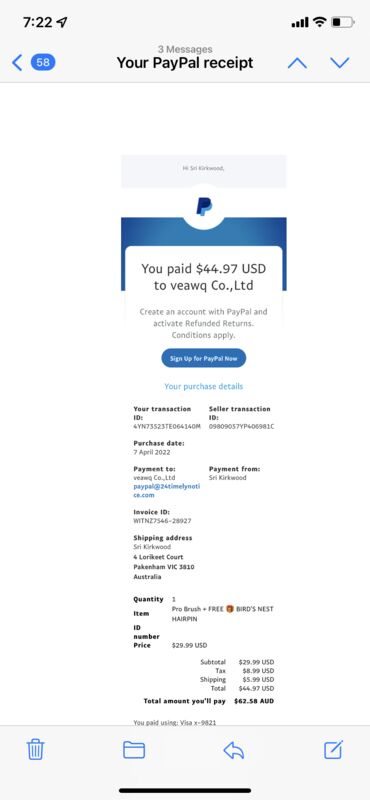The image captures a screenshot of a cell phone display showing a PayPal receipt. At the very top of the screen, typical mobile phone widgets are visible; these include the time on the top left, with it displaying "58" inside a blue circle, and on the top right, icons indicating signal strength, WiFi connectivity, and battery status – the battery is around half full.

Below the widgets, a header in the center reads "Your PayPal Receipt" in a prominent black font. Just above this in smaller gray text, it indicates there are "three messages." On the top right of the header, there are up and down caret arrows, while on the top left, there is a left-facing caret.

Directly under the header, the PayPal logo is prominently featured in the center, followed by a blue header that aligns with PayPal's signature design. The text below the header states, "You paid $44.97 USD to veawqco.ltd." This section is accompanied by additional text which likely contains transaction details, and a large blue button underneath.

Continuing downwards, the receipt extends to provide more specific details of the transaction including payment address, payer, and payee information.

At the bottom, a footer bar offers various options with icons for trash, file, send, and compose.